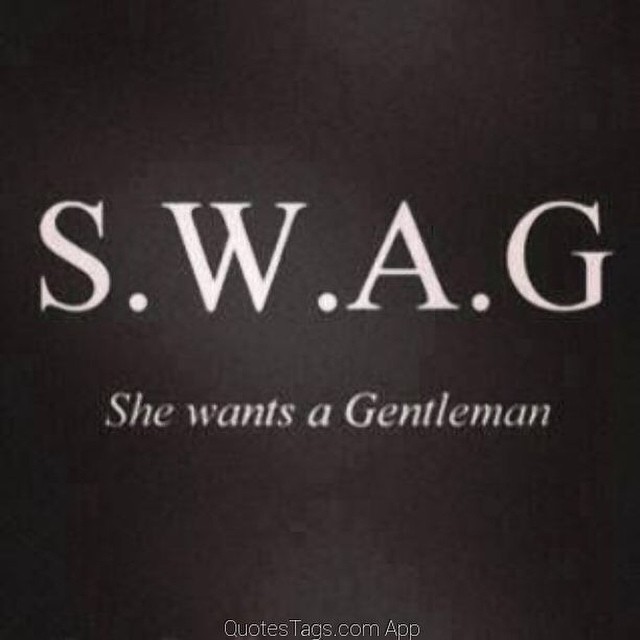This image, resembling a vintage meme commonly found on social media, features a grainy black background that fades to a lighter gray towards the center, giving it a slightly blurry and aged appearance. Dominating the upper half of the image in large white letters are the initials "S.W.A.G." written with periods after each letter. Just below this acronym, in smaller white text, is the phrase "she wants a gentleman," where "gentleman" is capitalized. At the very bottom of the image, in thin white letters, the text reads "QuotesTags.com app," marking it as likely an advertisement.